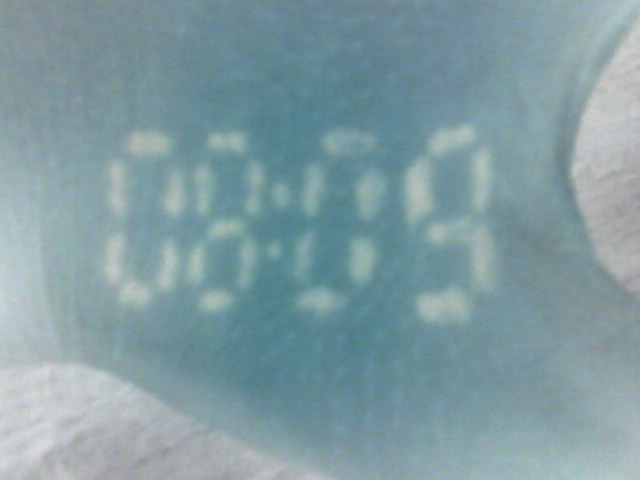A heavily blurred image featuring four indistinct numbers in the style of a digital clock display, reading "08:09." The background is nondescript, with the focus entirely on these numbers. The graininess and out-of-focus quality make it challenging to discern any further details.